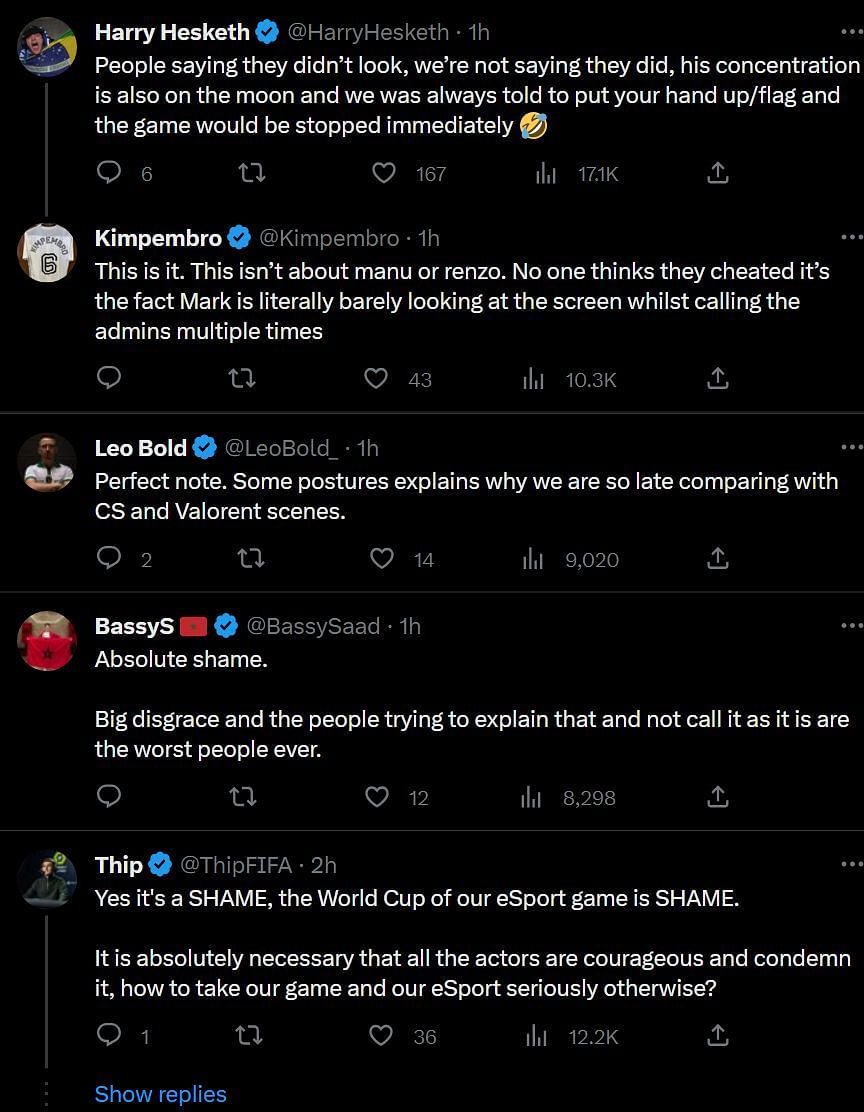Here is the detailed description of the Twitter conversation:

---

**Screenshot of a Twitter Conversation:**

The image is a screenshot of multiple interactions on Twitter, prominently featuring verified users. 

1. **Harry Hex Keith (verified)** (@HarryHexKeith) - **1 hour ago:**
   - "People saying they didn't look, we're not saying they did. His concentration is also on the moon and we've always told you to put your hands up/flag. And the game wouldn't be stopped immediately 😂"

2. **Kimp (verified)** (@KIMPENBRO) - In response to Harry Hex Keith:
   - "That is it. This isn't about Manu or Renzo. No one thinks they cheated. It's about the fact that Mark is barely looking at the screen while calling the admins multiple times."

Below this interaction, various other verified users contribute to the discussion:

3. **Leo Bold (verified)** (@PerfectNote):
   - "Some postures explain why they were so late with comparing CS and Valorant scenes."

4. **Bassy S (verified)** (@BassyS) - Accompanied by a red emoji:
   - "Absolute shame, big disgrace. And people trying to explain that and not call it as it is are the worst people ever."

5. **Thip (verified)** (@Thip) - In all caps:
   - "YES, IT'S A SHAME. THE WORLD CUP OF OUR E-SPORT IS A SHAME. It is absolutely necessary that all the actors are courageous and condemn it. How can we take our game and our e-sport so seriously otherwise?"

---

The conversation centers on an apparent controversy involving focus and integrity during an unspecified e-sport event, with multiple verified individuals voicing their concerns and criticisms regarding the conduct displayed.